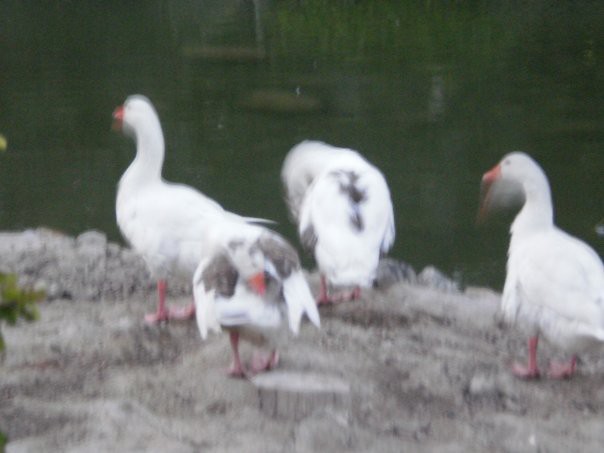A slightly blurry color photograph captures four white geese with orange beaks and feet, standing on a rocky and grayish dirt surface scattered with a few stones and dry twigs. Two of the geese feature gray markings on their backs, distinguishing them from the other two, which are entirely white. The geese are all walking away from the camera toward the back left of the image, with two partially bent over, making their heads less visible. One goose appears to be preening its tail feathers. The background is a mix of murky dark green, possibly indicating vegetation, and there is visual ambiguity suggesting a nearby body of water, potentially a pond. The image may include the faint outline of a building and some plant life on the left edge. The photograph conveys a sense of motion, as the geese seem to be in mid-step.